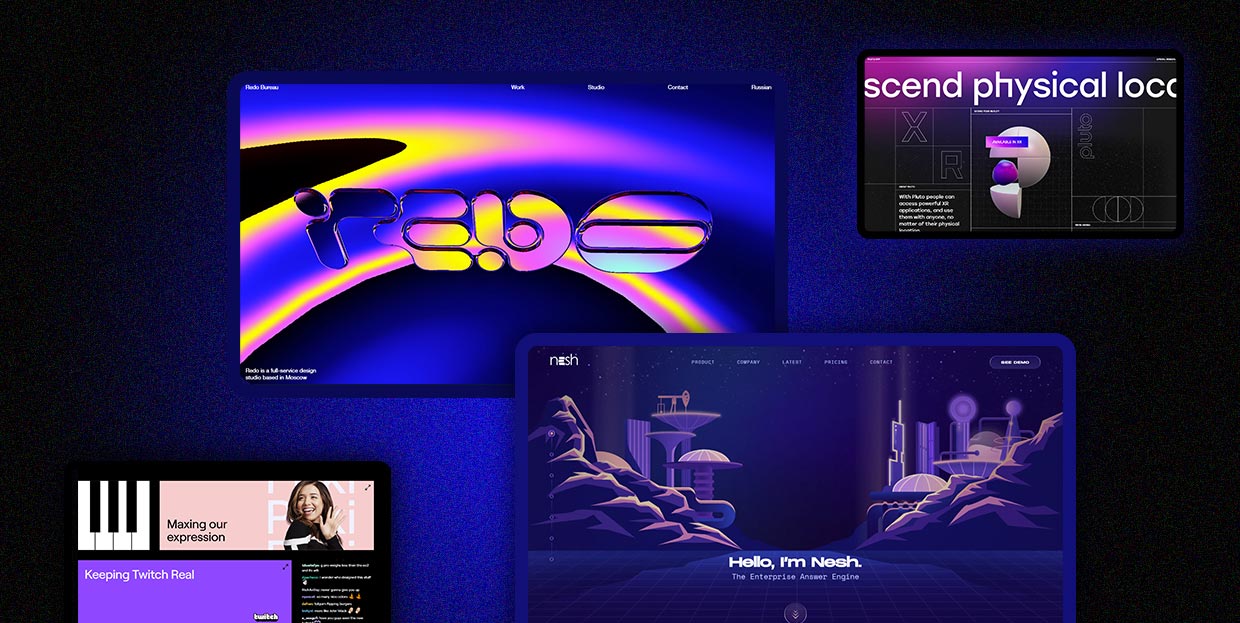The image resembles a TV screen divided into four sections, each containing distinct elements. The upper right quadrant features a slightly smaller square with the partial text "S-C-E-N-D physical L-O-C-O" and a Pac-Man-like symbol at its center. In the middle of the screen, there are two overlapping squares: one positioned towards the upper left and the other slightly below, overlapping the lower right corner of the square above it. The lower left quadrant contains a smaller square, completing the sporadic arrangement of these four sections. Each square seems to depict unique content, creating a composite visual layout.